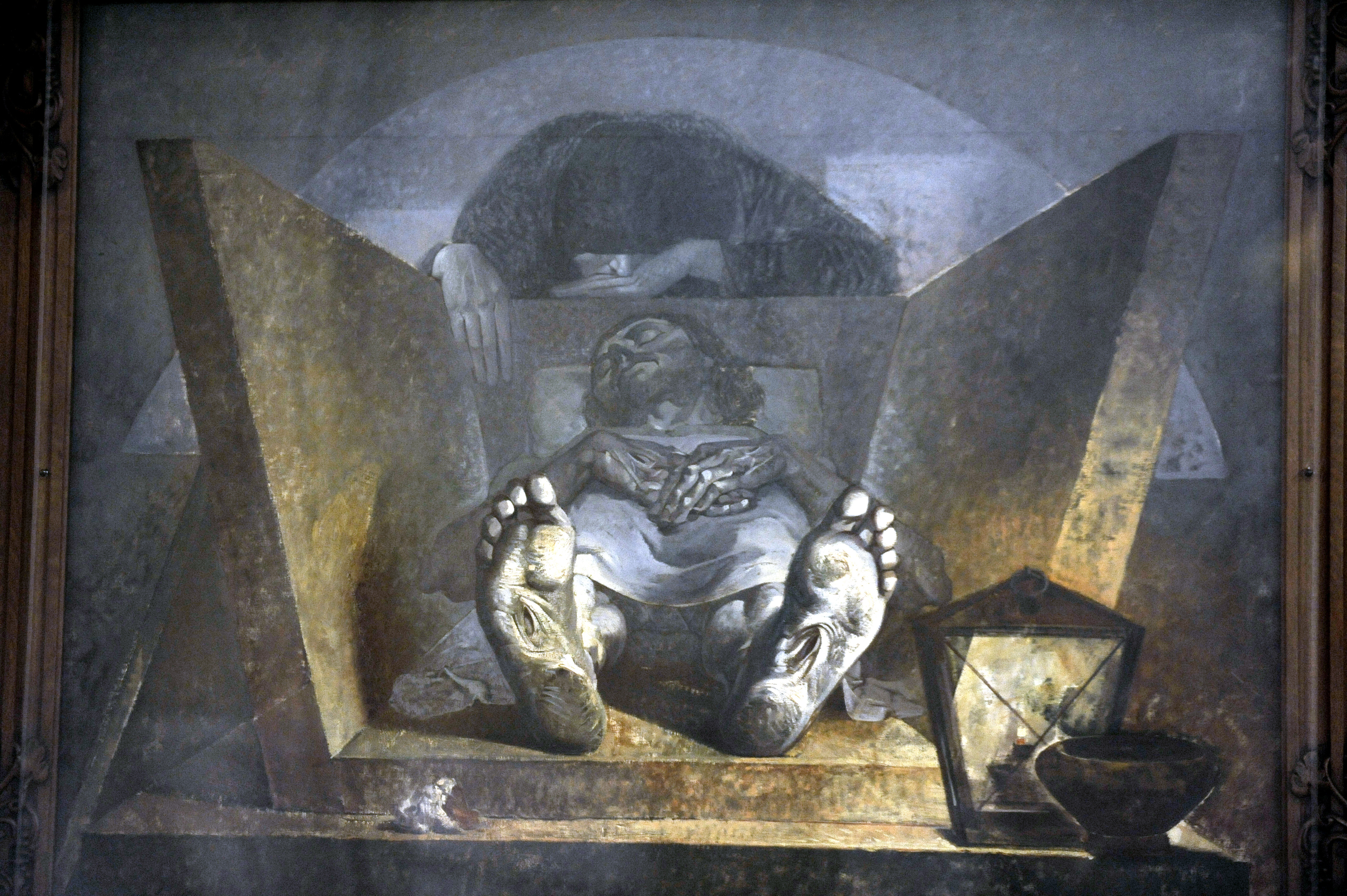This intricate painting depicts a solemn and morbid scene centered around a deceased man lying in an open tomb or coffin-like structure. The man, who bears a resemblance to Christ, has grayish skin with puncture-like marks visible on the bottoms of his bare feet. His arms are crossed over his chest, and he wears a white robe, enhancing the lifeless and somber tone of the artwork. Above him stands a figure cloaked in a black robe, presumably a woman, whose face is partially obscured by a shroud, revealing only her nose and part of her lips. Her posture and hand placement convey a deep sense of melancholy as she looks downcast, with one hand resting on the edge of the tomb and the other hand near her face.

The surroundings consist of cold, gray stonework with hints of blue, contributing to the gothic atmosphere of the scene. In the foreground, a lantern and a small bowl, both brown, sit near the open-bottomed coffin, providing the only sources of light and emphasizing the darkness of the setting. The overall mood is one of solemnity and reflection, accentuated by the shadowy and somber colors throughout the painting.